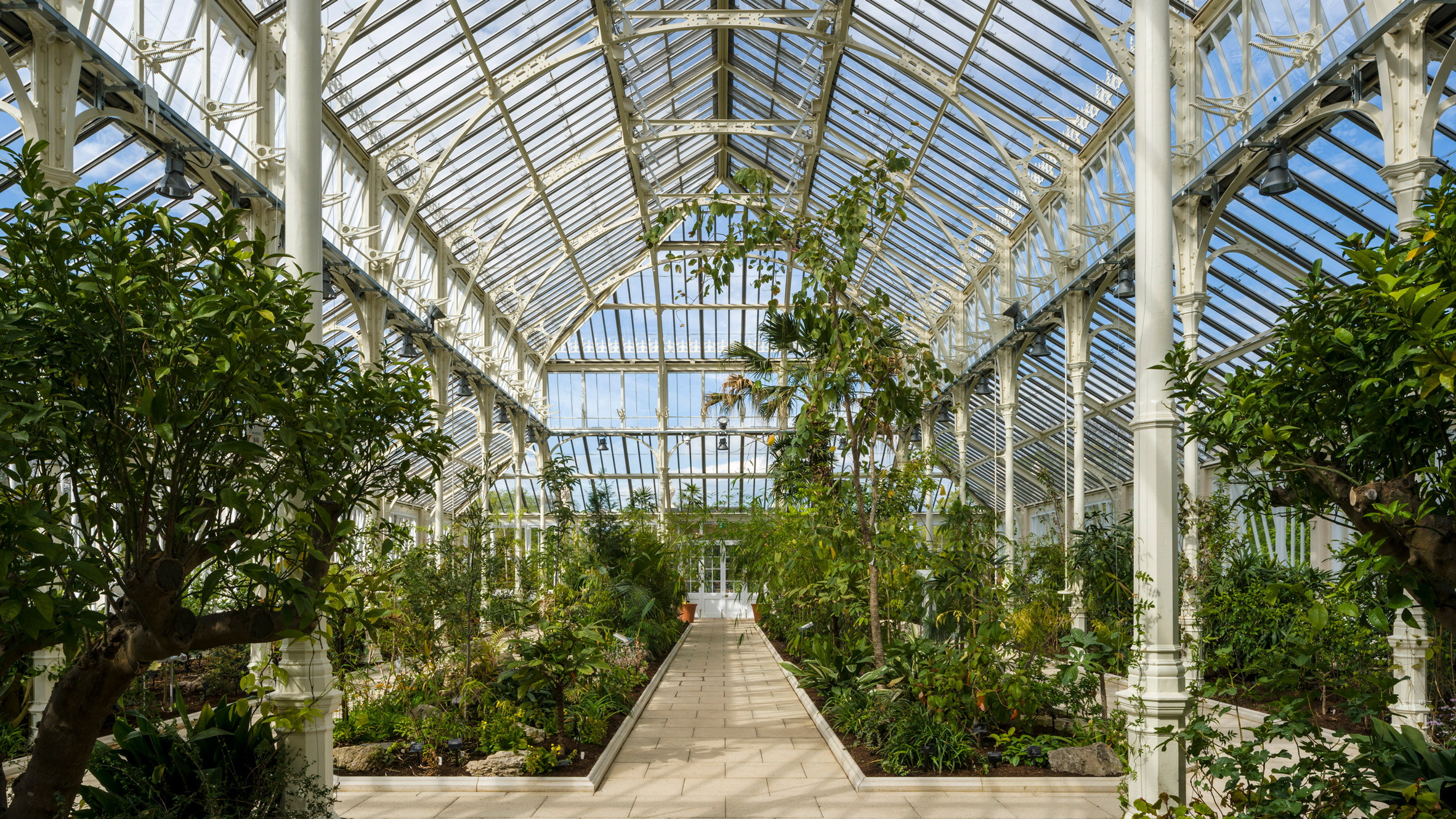The photograph captures the interior of a large greenhouse, characterized by its towering structure composed of white-painted steel and transparent glass panes. The clear glass ceiling offers a picturesque view of a slightly cloudy blue sky, allowing abundant natural light to flood the space. Inside, the ground features walkways made of cream-colored rectangular bricks or tiles, forming pathways between the various plants. These plants, which include an array of small shrubs, green bushes, and several slender trees with brown trunks and green leaves, line both sides of the greenhouse, creating a lush, verdant environment.